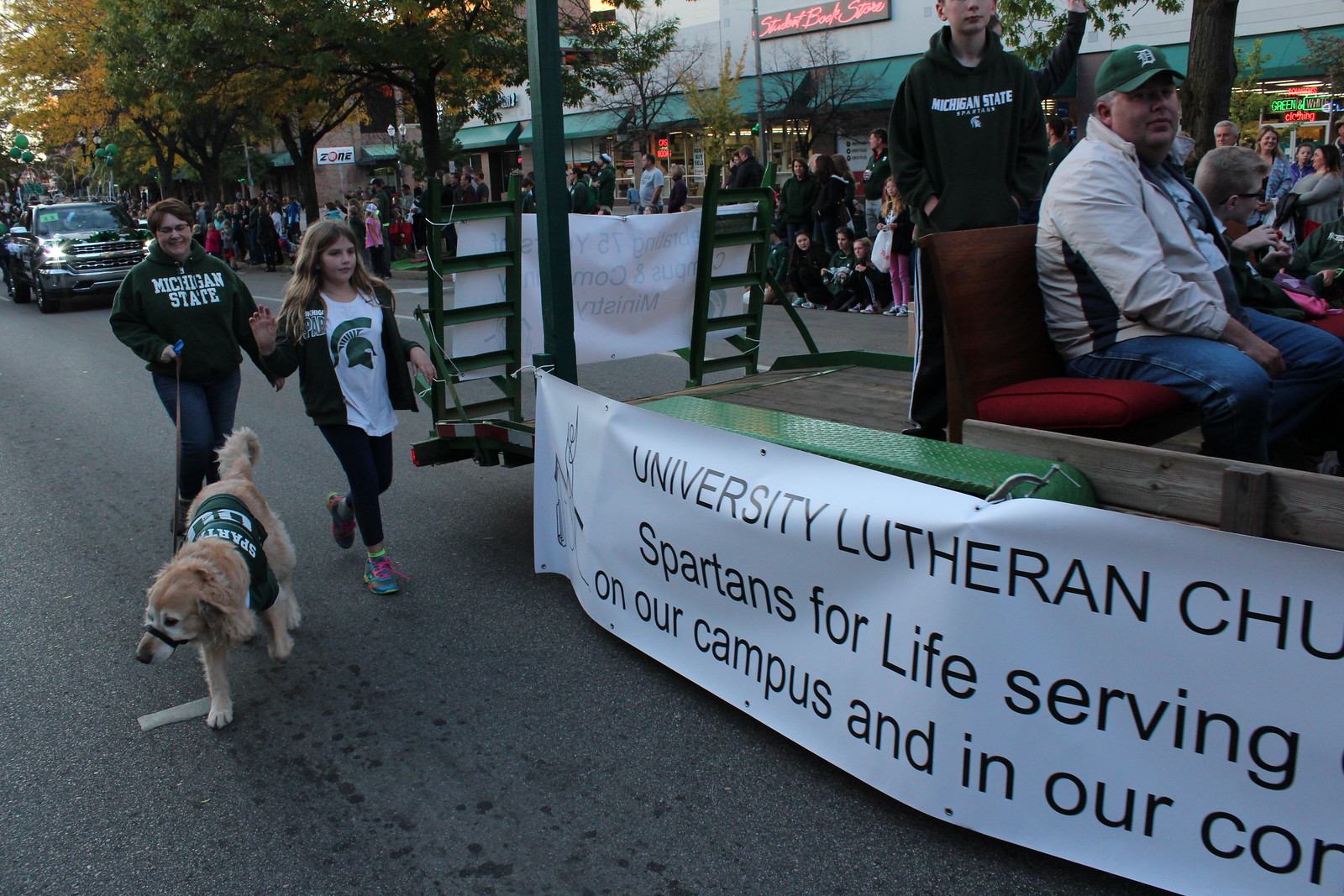This vivid color photograph captures a bustling outdoor parade, where a float representing the University Lutheran Church takes center stage. The float proudly displays a white banner with black lettering that reads, "University Lutheran Church Spartans for Life serving on our campus and in our community," though part of the message is cut off. Seated on the float is a man in his 50s, clad in a white jacket, blue jeans, and a green ball cap. Beside him is a young man standing in a black sweatshirt with a white graphic, though his head is partially out of frame. 

Behind the float, a young girl and her mother, both in Michigan State attire, walk hand-in-hand, accompanied by a golden retriever dressed in green Spartans gear. The background reveals a truck adorned with green balloons and a lively crowd of approximately 100 people lining the street, eagerly watching the parade. The scene is set against a backdrop of city shops, capturing the vibrant essence of community celebration. The style of the photograph is a realistic representation, providing a detailed and immersive view of the event.